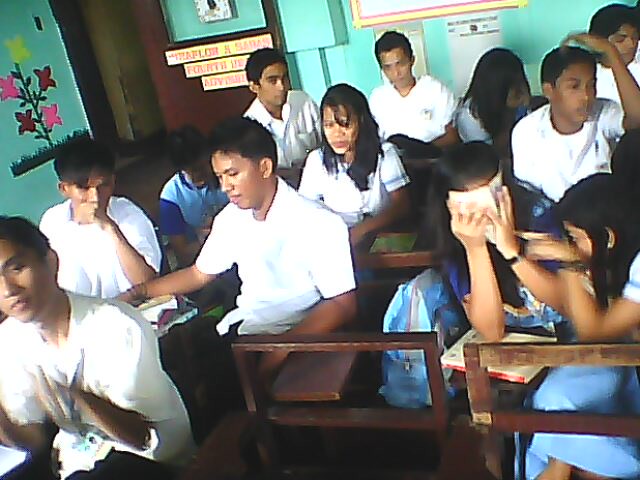The image captures a bustling classroom filled with older children, likely high school or college students. The room is decorated with soothing light greenish-blue walls and features a mural of a plant with green stems and yellow, pink, and brown flowers growing from flat grass, positioned on the upper left corner. The students are seated closely together in brown, squared wooden chairs that have built-in desk surfaces. The majority of the students are wearing white shirts, although there are notable exceptions, such as a girl in a blue and white dress, and another student in a blue shirt with an animal design, who has a black wristband and is holding a yellow booklet to her face. A blue and purple backpack is visible between two students at the front. The photograph also reveals an open brown door with a window situated at the back corner of the room. Additionally, the image includes some unreadable signs with red lettering on the back wall and door. The atmosphere appears crowded and slightly blurry, but distinctly captures the vibrant, youthful environment of the Southeast Asian classroom.